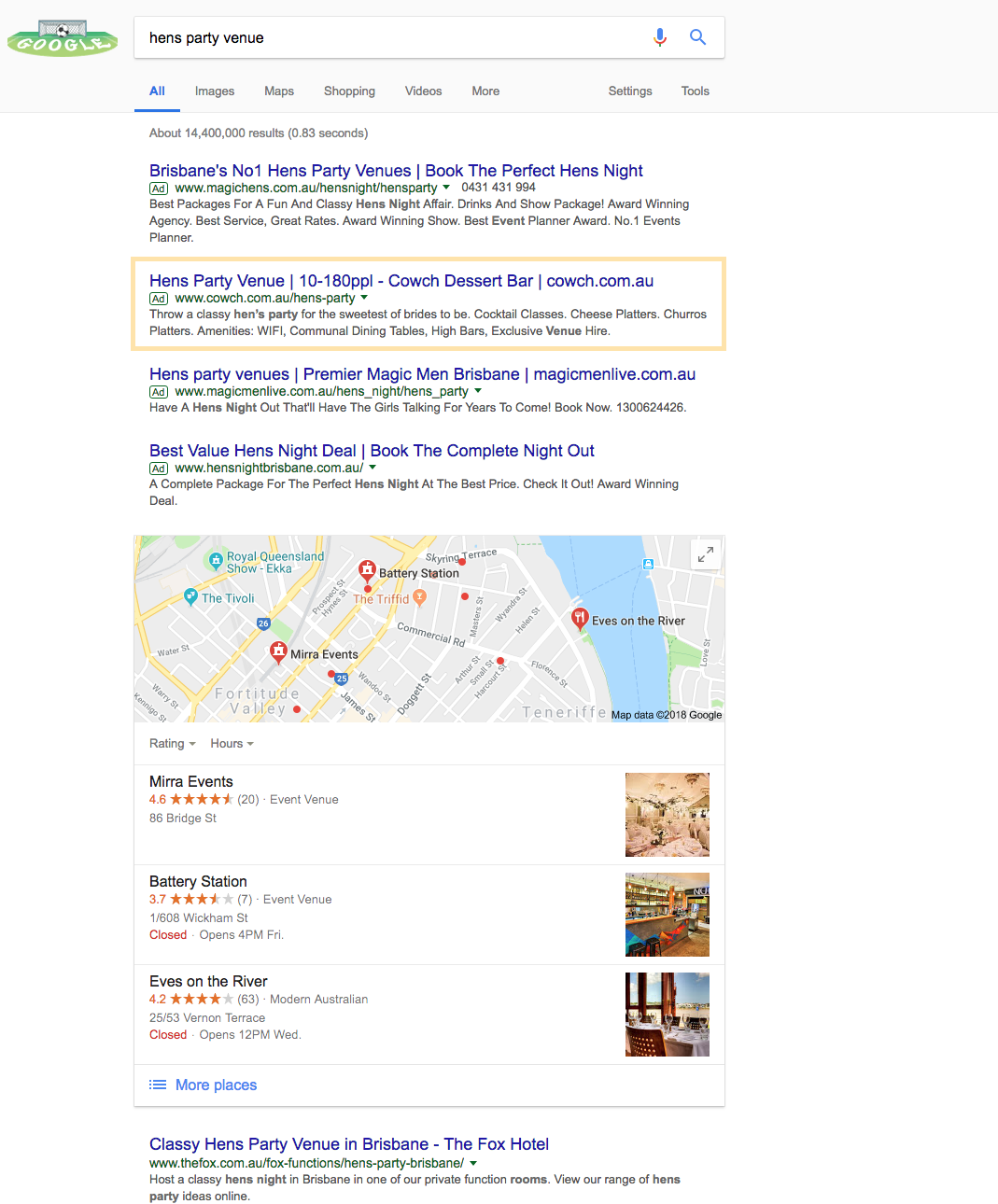A search result page from a website is displayed. At the top of the page, a gray search bar contains the text "Ken's party venue" written in black. Below the search bar, four paragraphs are displayed with their top lines highlighted in blue, while the remaining text is in black. The second paragraph is emphasized by being enclosed within a light orange rectangle. 

A map is also visible on the page, marked with red pinpoints indicating various locations. Beneath the map, on the left side, text is displayed listing "Events," "Battery Station," "Eaves on the River," and what appears to be "Mira Events" or "Mire Events." Adjacent to the text descriptions are small photos, though their details are difficult to discern due to their size.